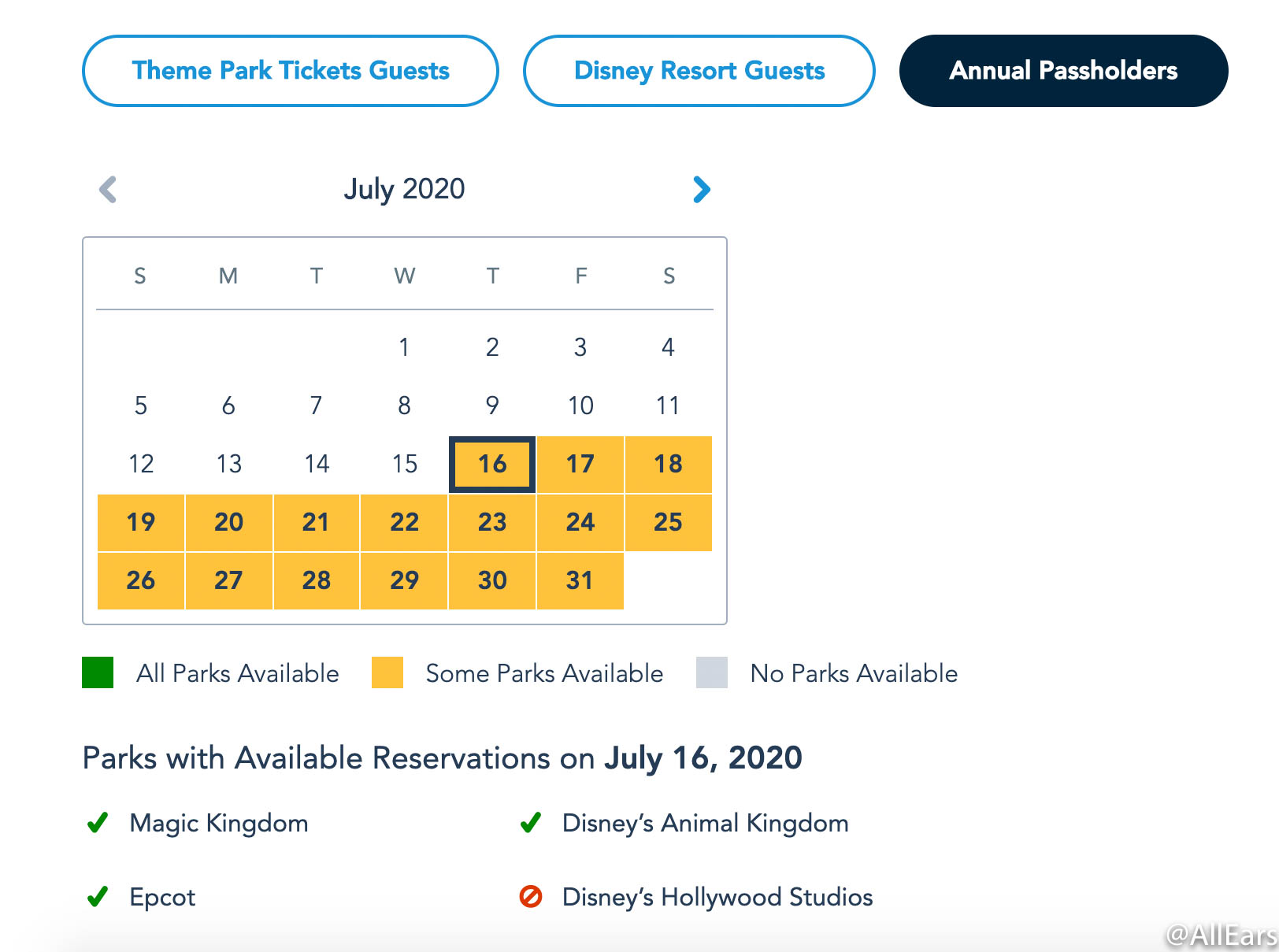This image appears to be a screenshot of a reservation system within a Disney-themed or calendar application. At the top, three pill-shaped buttons are prominently displayed. The first two buttons feature a light blue outline with light blue text on a white background, labeled "Theme Park Ticket Guests" and "Disney Resort Guests." The third button displays "Annual Pass Holders" in white text on a solid dark blue background.

Beneath these buttons, there is a calendar for July 2020. Navigation arrows allow the user to move between months. The calendar grid distinctly highlights the dates from the 16th to the 31st in yellow, indicating dates with limited park availability. The 16th is further emphasized with a square outline, suggesting it is the current date.

A legend below the calendar clarifies the color-coding: green signifies full park availability, yellow indicates partial park availability, and gray denotes no availability.

Under this key, specific information about park availability for July 16, 2020, is provided. Magic Kingdom, Epcot, and Disney's Animal Kingdom all have a green check mark, indicating availability. Disney's Hollywood Studios, however, has a red bar with a diagonal slash, denoting no available reservations.

In the lower right-hand corner, there is an "Add All Ears" text icon with a drop shadow, placed against a clean white background. This feature appears designed to assist users in booking tickets for Disney parks and attractions.

The overall functionality of the app seems to facilitate the reservation process for various Disney parks, ensuring guests can plan their visits efficiently based on real-time availability.